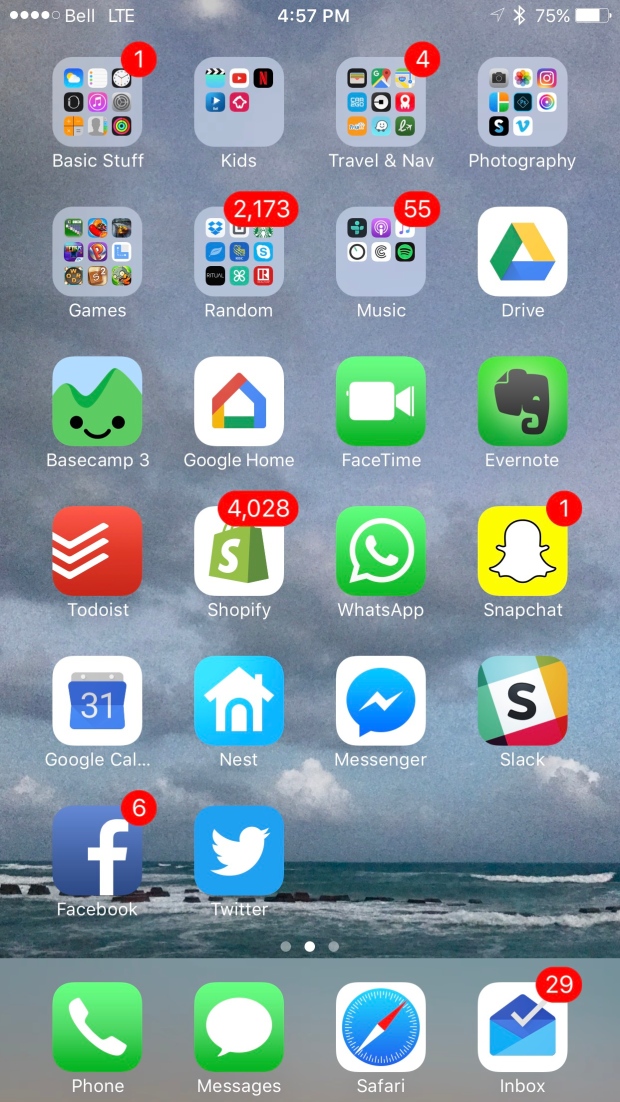The image features a Google smartphone screen showcasing a meticulously organized home screen layout. The apps are arranged into two distinct sections. 

The upper section comprises various categorized folders labeled "Basic Stuff," "Kids," "Travel & Navigation," "Photography," "Games," "Random," and "Music." Notably, the "Random" folder contains an astonishing 2,173 apps, the "Music" folder includes 55 apps, and the "Travel & Navigation" folder has four apps.

In the lower section, more commonly used Google apps and social media applications are laid out separately for convenience. These include Google Drive, Google Home, FaceTime, WhatsApp, Snapchat, Messenger, Slack, and Google Calendar. Some of these apps display notification indicators, such as Snapchat and Facebook, hinting at updates or unread messages. Specifically, the inbox icon reveals that there are 29 unread messages.

Interestingly, the Shopify app stands out with a striking 4,028 items, implying extensive activity, although the exact nature—whether buying or other—is unclear. 

Overall, the screen's organization exemplifies a user who prioritizes both categorization for specific tasks and quick accessibility to frequently used applications.